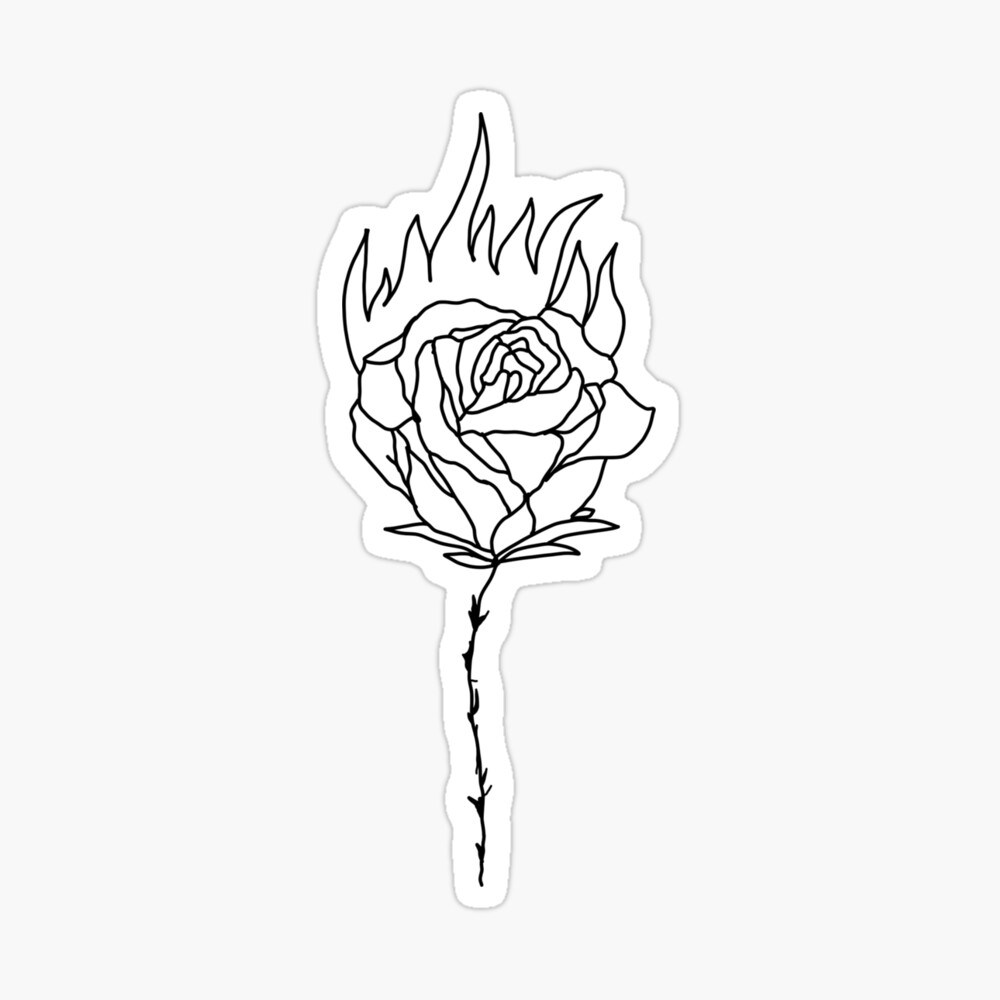The image is a black and white line drawing of a rose, depicted in a style reminiscent of tattoo flash art or a sticker. The rose, which is mostly in bloom, sits atop a thorny stem with several protruding thorns. Below the rose, there are a few small leaves. Above the topmost petals, flames or flame-like shapes extend upwards, adding a dramatic flair to the illustration. The entire drawing is set against a white background with a slightly off-white border, enhanced by a light gray drop shadow. The lines of the drawing are of uniform weight, contributing to the simplicity and clarity of the design.